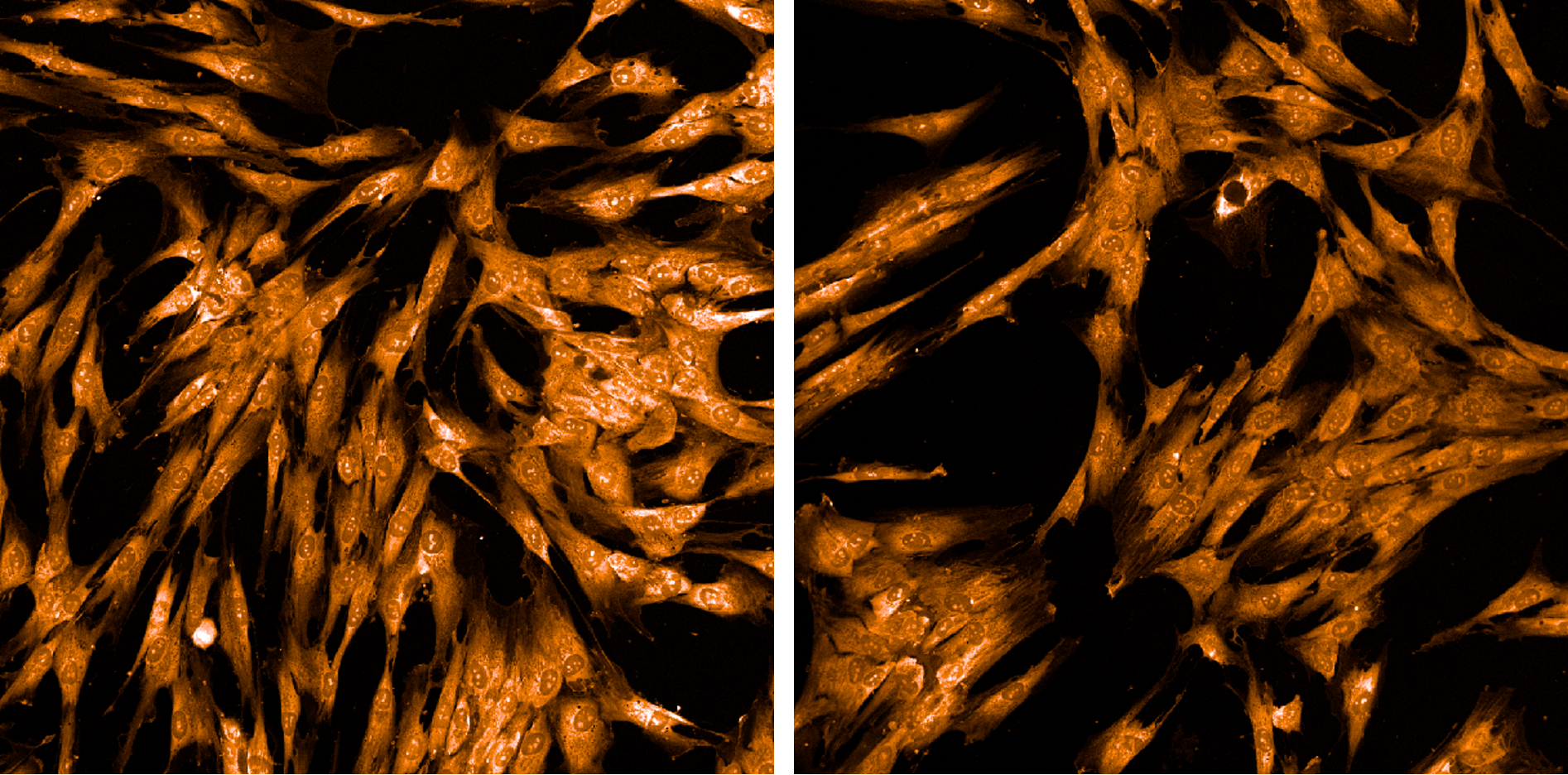The image consists of two side-by-side square visuals separated by a white bar. Both images feature a black background with dark orange-brown structures that appear like clusters of intricate, vein-like patterns. These plasma-like forms are numerous and interconnected, resembling either a close-up of plant cellular structures or clusters of small, fish-like creatures. Despite their dense arrangement on the left side, they are more sparsely distributed on the right, giving a sense of dynamic flow and organic design. Overall, the images evoke an artistic, almost microscopic perspective, emphasized by repeating patterns and the stark contrast between the vibrant orange-brown elements and the solid black backdrop.